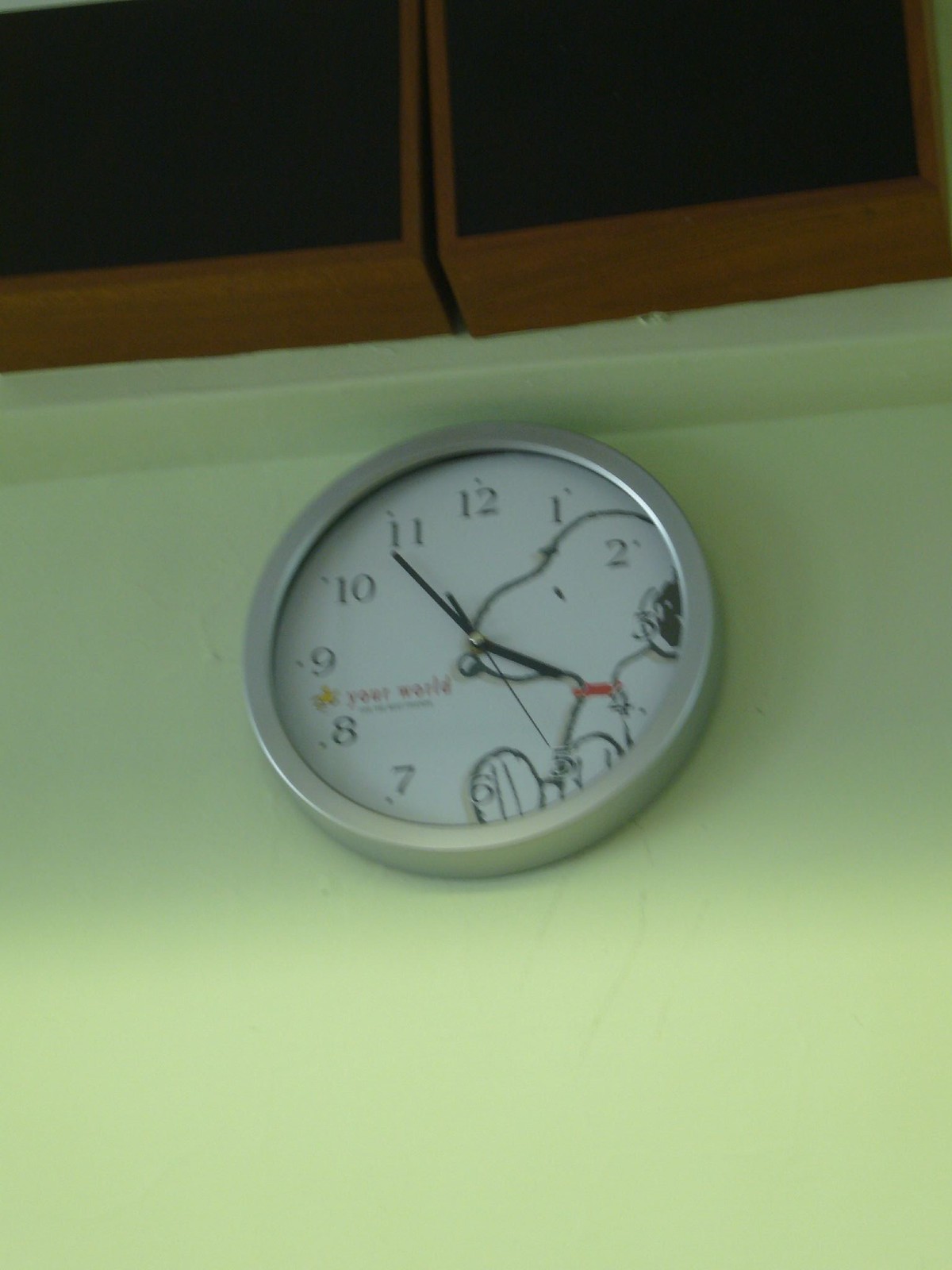This indoor color photograph, taken from a slight upward angle, showcases a round wall clock mounted on a pale green wall. The wall clock features a silver bezel and a white face adorned with a profile image of Snoopy from the Peanuts comic strip, illustrated in black and white with a red collar. Snoopy is positioned to the right of the clock's center, gazing down towards the clock hands, which are all black. The clock also includes black numerals from 1 to 12, and a small depiction of Woodstock, represented by a yellow dot, is located between the 8 and 9. To the right of Woodstock, the phrase "your world" is written in red lettering. Above the clock, two rectangular wall-mounted speakers with either green or black grills and dark brown wooden casings are affixed horizontally. The upper portion of the image is slightly out of focus and shadowed, with the lower part of the wall appearing lighter.